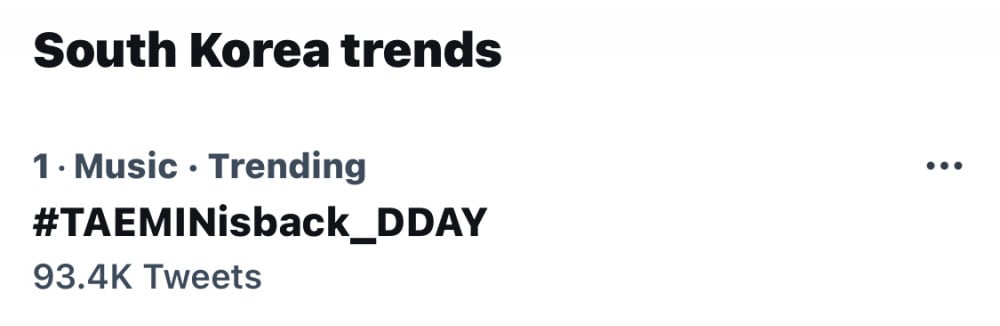The image features a digital card presented in landscape mode with a completely white background. It consists of four rows with distinct information:

1. In the top left corner, the phrase "South Korea Trends" is bolded in large black font.
2. The second row contains the number "1", followed by bullet points separating the words "Music" and "Trending" in gray text. On the right side of this row, there are three vertically arranged dots, presumably an icon for additional options.
3. The third row highlights "#TAEMIN_is_back_D-Day" in bold black font, signifying a trending topic. Below this, the text "93.4K Tweets" indicates that approximately 93,400 tweets mention this hashtag.
4. The caption hypothesizes that TAEMIN is likely a South Korean musician, singer, or performer, stirring significant excitement among users, as reflected by the high tweet count, making it a trending topic in the Music category in South Korea.

This highly detailed and organized presentation of trending data underscores the fervent social media activity surrounding the topic of TAEMIN's return.